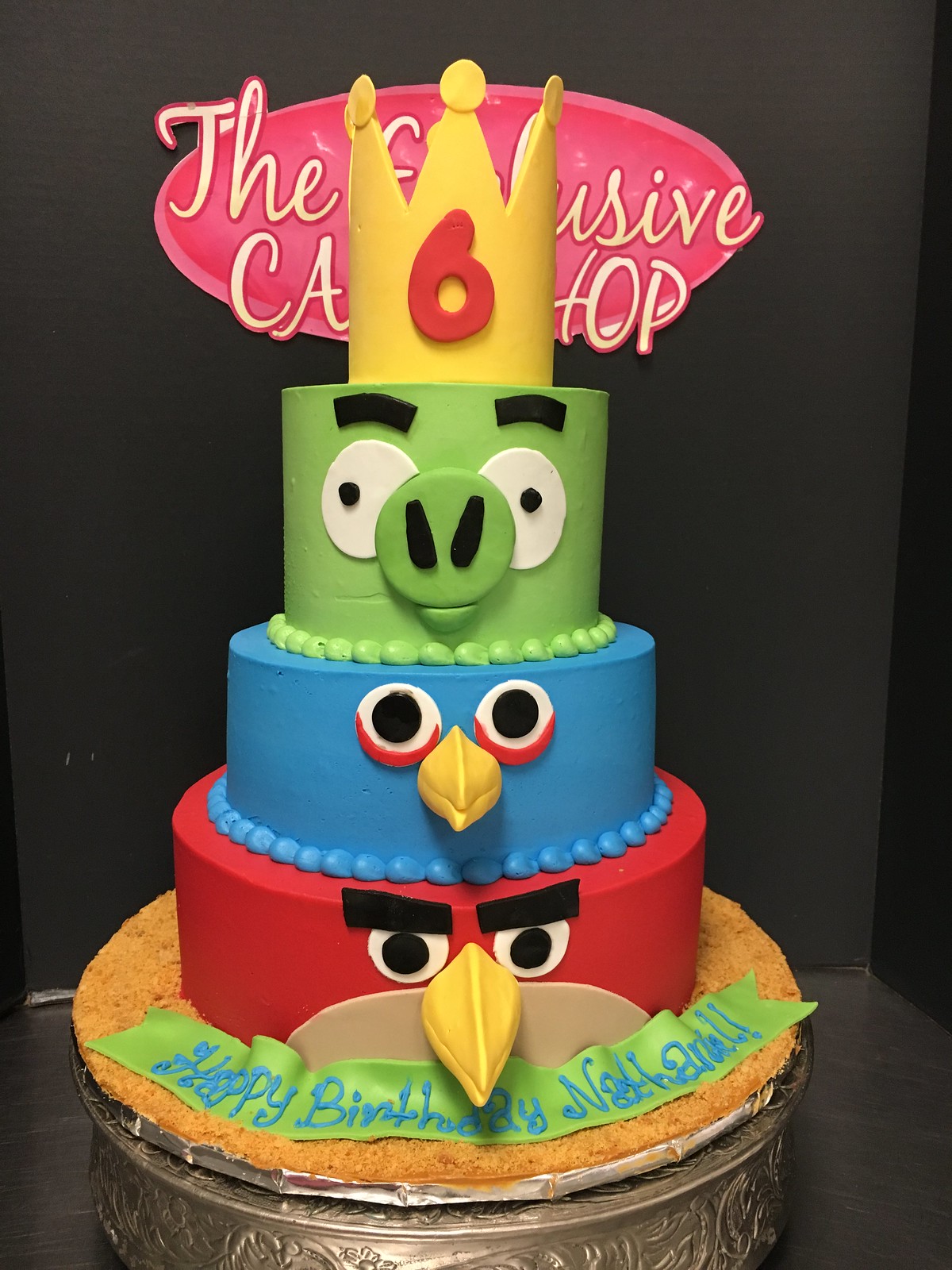This is a color photograph of a creatively designed birthday cake for Nathaniel, set against a matte black background. The cake stands tall with four distinct tiers adorned with characters from the iconic Angry Birds game. At the very base, it features a metallic decorative base or foil lining. Just above this base, a green ribbon banner reads "Happy Birthday Nathaniel!" in blue lettering. 

The first tier showcases the Red Angry Bird with a yellow beak, white eyes, and angry eyebrows. Above this, the second tier displays the Blue Bird, characterized by red bags under its eyes and a yellow beak. The third tier features the Green Pig, complete with a green snout, black nostrils, wide white eyes, and thick dark eyebrows giving a slightly surprised expression. 

Crowning the cake is a yellow crown with a red number six on the front. Behind the crown, partially obscured, is a pink oval logo with lighter pink bordering, possibly belonging to the cake shop. The visible parts of the logo read bits and pieces like "THE," "USIVE," and "CAPITALS C A HOP". The intricate details and vibrant colors make this cake a delightful centerpiece for Nathaniel's birthday celebration.